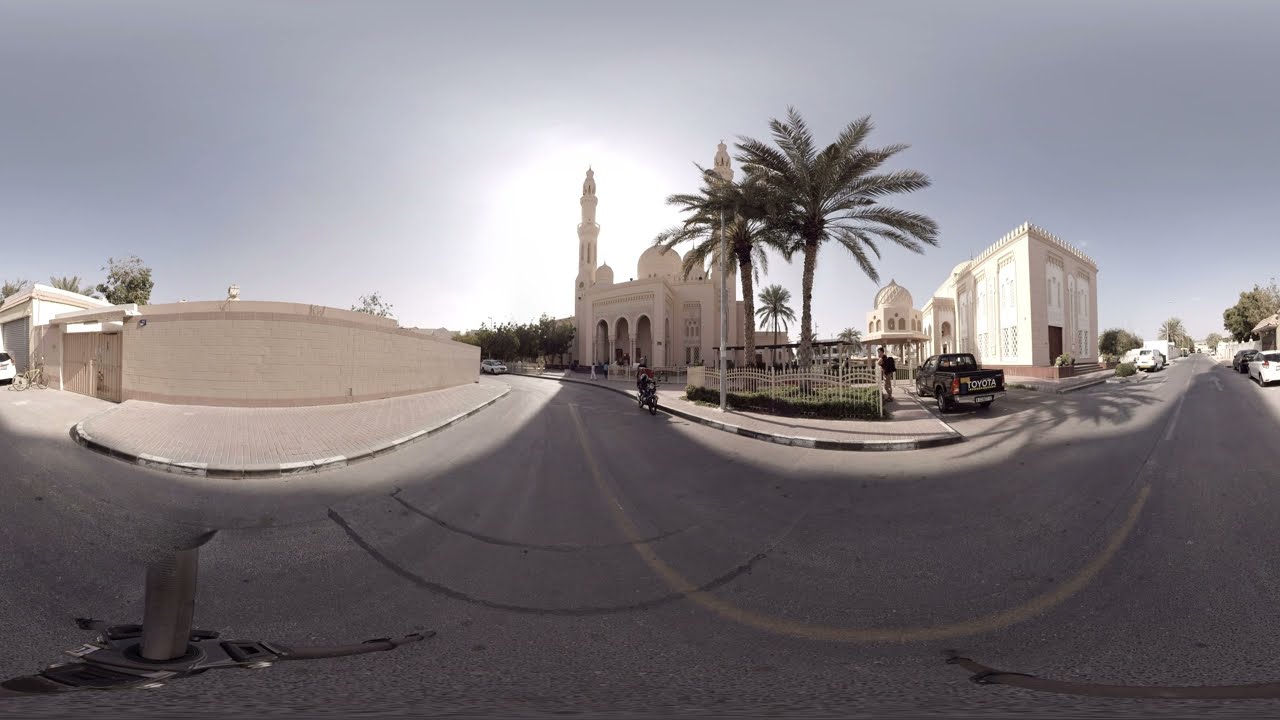The image captures a visually striking street scene, distorted by a fisheye or panoramic lens, adding a unique curvature to the perspective. The main street runs from the right side to the center, featuring a light-gray pavement with a faintly visible yellow line that curves gently towards the middle. Cast in varying shades of shadow, the street is lined with distinctive buildings. On the right, there's a tall, white building with an arch on top, accompanied by a narrow and tall palm tree, its fronds extending in all directions. Adjacent to this building, a dark Toyota pickup truck is parked next to the curb, with a man standing beside it, close to a metal and wooden barrier that encloses some vegetation.

To the left of the white building, another structure with steep, pointed steeples rises sharply into the sky. In front of it, a person on a motorcycle or moped, possibly wearing something red, rides along the curb. Further left stands a flat light-brown building with darker trim, partially hiding another white-colored structure, in front of which a white vehicle is parked.

The background reveals a sunlit sky, transitioning from a bright white center to a pinkish hue, with a light gray expanse on either side. Dotted throughout the scene are several cars, including another white vehicle and additional greenery in the form of palm trees. The overall atmosphere is one of a bright, pleasant day, with the combination of architectural elements and natural features creating a richly detailed and somewhat surreal tableau.